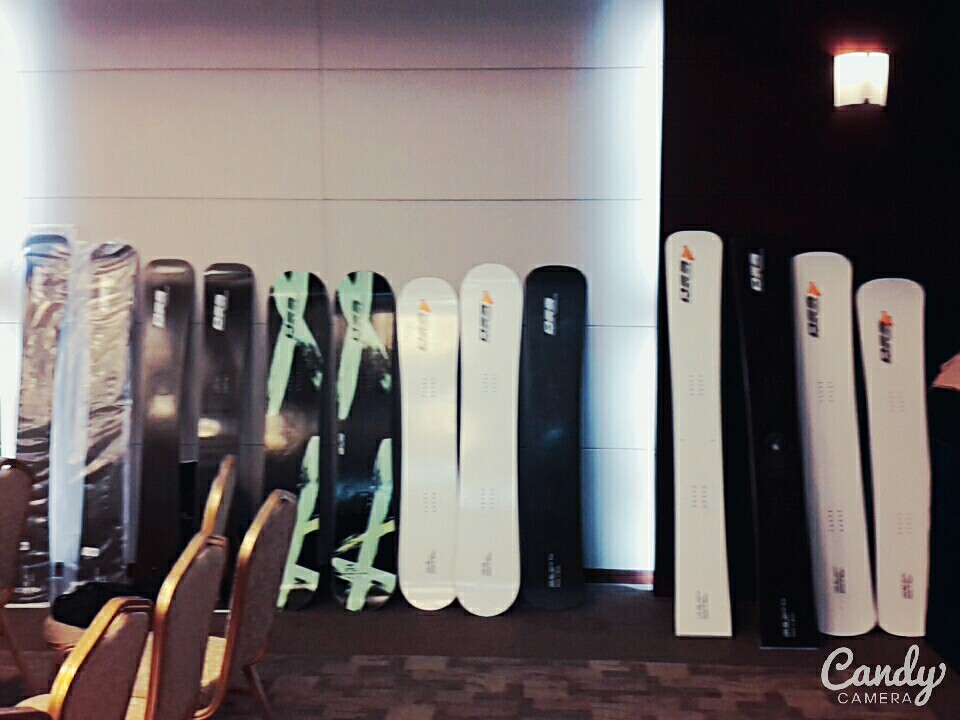In this somewhat blurry interior photo, an array of snowboards is vertically lined up against a white wall. The collection consists of various colors and patterns, predominantly featuring white and black boards. Notably, two of the snowboards exhibit black and lime green graffiti-like striping, while another displays a zebra pattern. The lower section of the image reveals four chairs positioned side by side, facing towards the left side of the frame. Additionally, the bottom right corner prominently displays the text "Candy Camera." The snowboards appear to be arranged in pairs, suggesting a matching set for each design. The scene is set against a brownish rug that contrasts subtly with the vibrant snowboard colors.